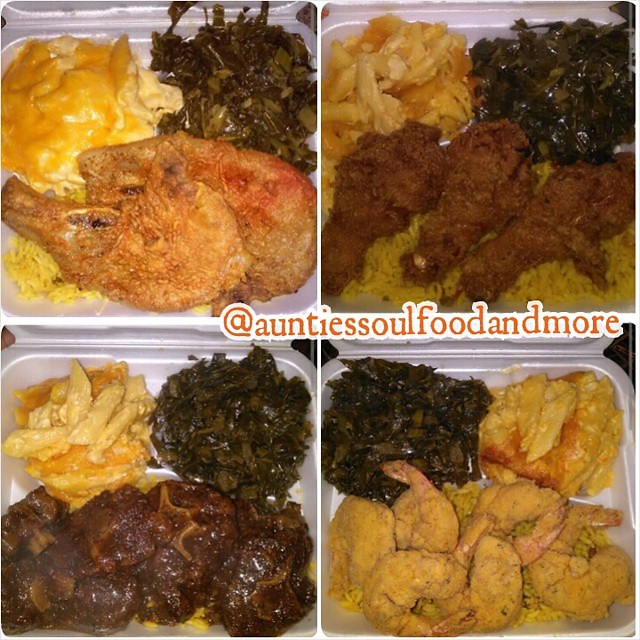This photograph is a collage of four color images, each showcasing a white styrofoam take-out container filled with large portions of various Southern-style foods. At the top left, the tray contains mac and cheese, collard greens, pork chops, and rice. The top right features mac and cheese, collard greens, fried chicken, and rice. The bottom left displays mac and cheese, collard greens, and a beef dish. The bottom right has mac and cheese, collard greens, and breaded shrimp. Each tray is densely packed, indicating hearty servings. A watermark reading "@auntie's soul food and more" is visible, slightly off-center to the right, across the images.